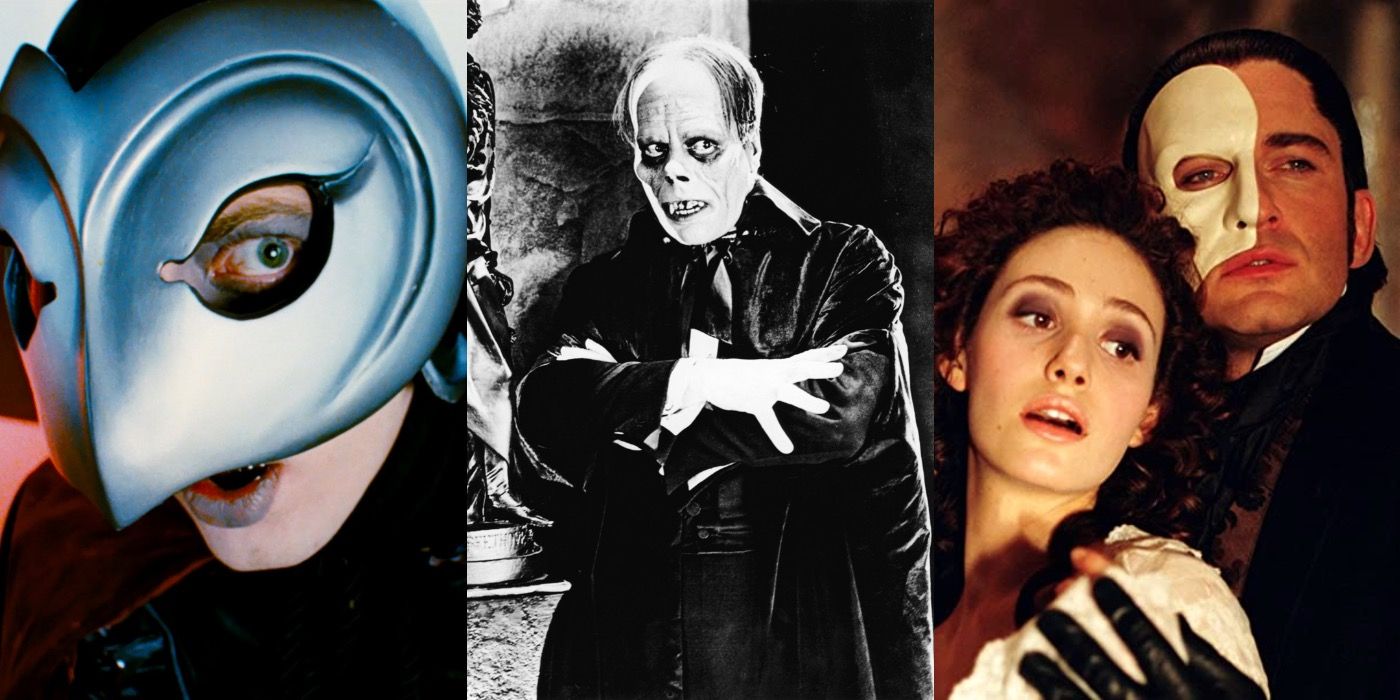This composite color image features three distinct interpretations of the Phantom of the Opera. On the far left is an image from Brian De Palma's *Phantom of the Paradise,* depicting a character with a beak-like mask, exposing one blue eye and pale blue lips, conveying a shocked expression. The central black and white photograph shows Lon Chaney's iconic portrayal of the Phantom, with dark rings under his eyes, an overlarge forehead with wrinkles, ghoulish fangs, and bad teeth. His right hand is raised dramatically as he gazes to the side. On the right, a more recent film adaptation portrays the Phantom standing behind Christine. The Phantom wears a white half mask, with his left hand, in a black glove, resting on Christine's shoulder. Christine, dressed in a white top with dark eye makeup, looks off into the distance, mirroring the Phantom's gaze. The varying interpretations across the three images capture the evolution of this enigmatic character.